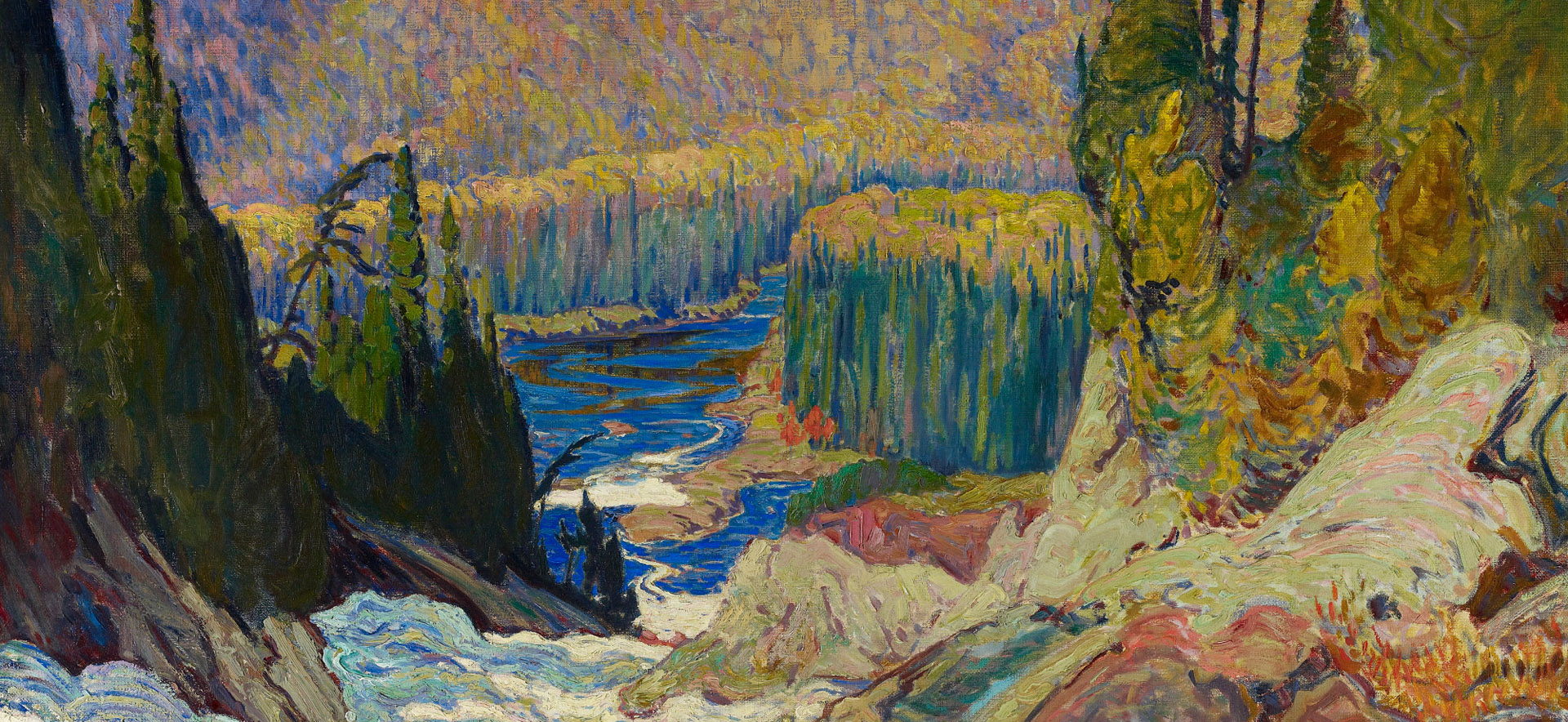This painting presents an abstract, impressionistic interpretation of a natural scene, blending elements reminiscent of both Claude Monet and Vincent van Gogh. The artwork captures a panoramic view, framed as a long rectangle. In the foreground, tall trees—potentially pines—and distinctive winding lines evoke van Gogh’s signature style, adding a dynamic sense of movement. There's a cascading waterfall flowing down a hillside, feeding into a stream or river that winds through a marshy area filled with tall grasses and cattails.

The background features a distant hill, covered with a mix of green trees and erosion marks, creating a sense of depth and perspective. Abstract elements, such as swirling strokes and vibrant colors, transform familiar natural features like rocks, yellow and orange blossoms, green leafy bushes, and clusters of colored rocks into a dream-like, almost surreal landscape. The depiction of water, with its blue hues and black swirls, contrasts against the yellow field of tall flowers, adding to the vibrant and interpretive essence of the scene. This painting eloquently blends natural beauty with artistic abstraction, offering a richly detailed and emotive representation of a nature scene.